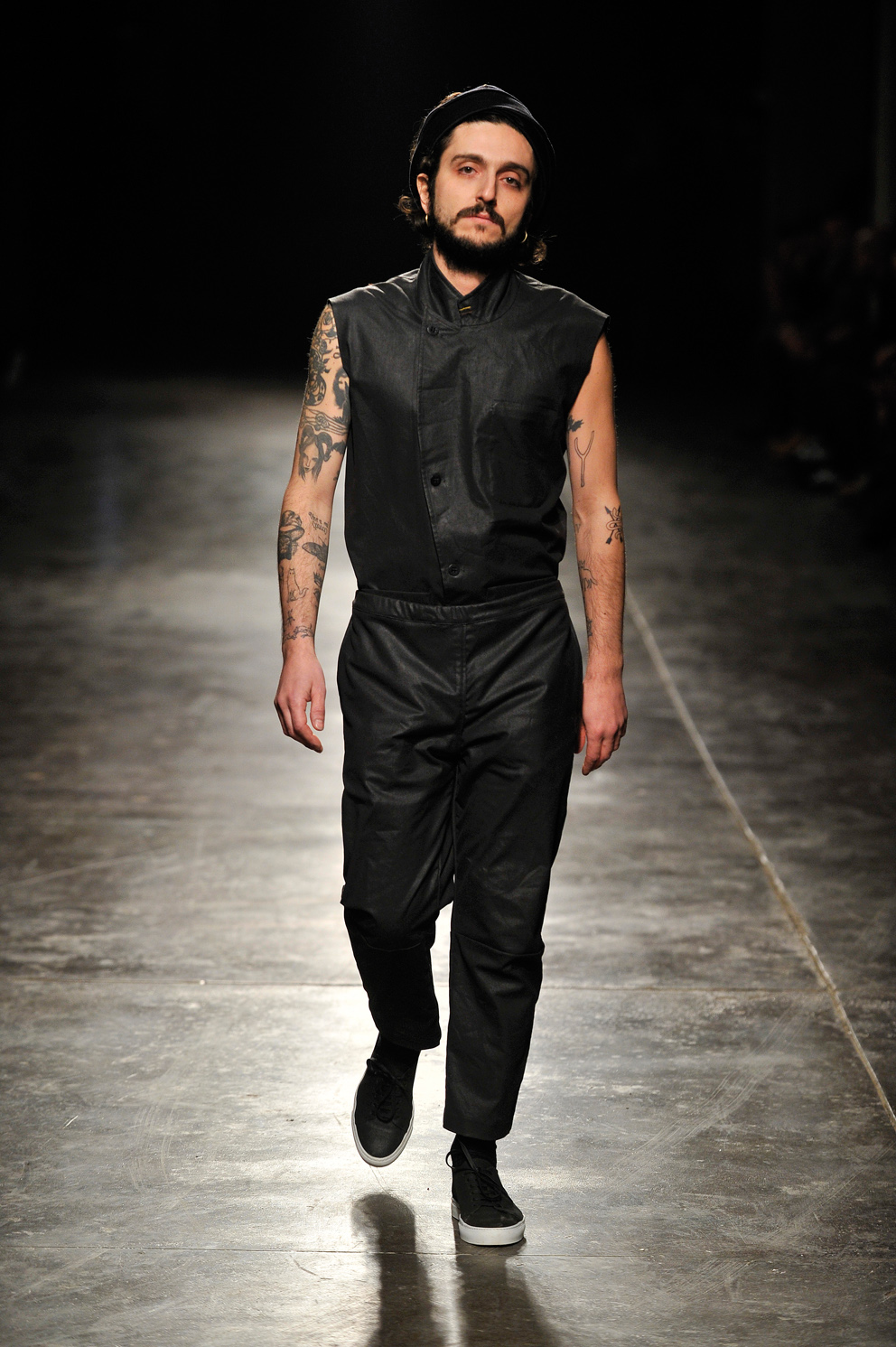In this striking image, a young man is captured walking down what appears to be a dimly lit runway or catwalk. The background is completely dark, illuminated only by a mysterious light source behind him, creating a dramatic silhouette. The man is dressed entirely in black, from his beanie-style cap to his high-topped sneakers with white soles. His attire includes shiny black pants that stop at his ankles and a sleeveless, collared button-up shirt with three buttons, both made from a fabric that catches the light with a subtle sheen.

He has a neatly manicured beard and mustache, dark hair, and a pair of silver earrings. His slender nose and green eyes stand out against his dark eyebrows. The man's arms are a canvas of tattoos: on his left arm, a wishbone tattoo on his bicep accompanied by other intricate designs, while his right arm features an array of tattoos including images of cats, a woman's face, and various symbols.

The runway or stage he is walking on has a shiny, black surface that contrasts with the nearly invisible, shadowy background, casting the man in a sharp, stylish light reminiscent of a fashion model on a high-fashion catwalk.